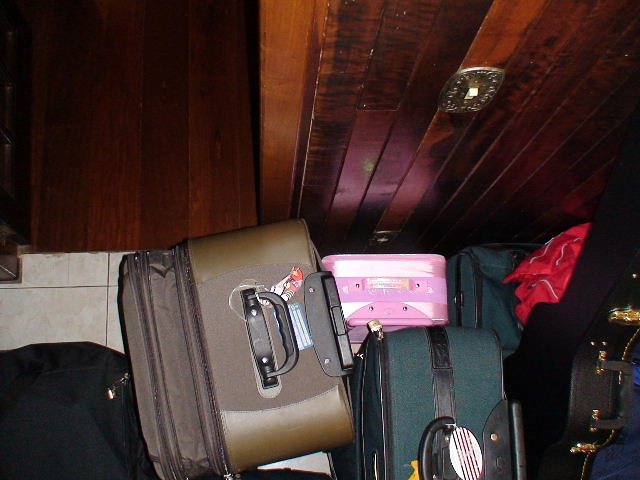The image presents an aerial view of a room or closet featuring a variety of suitcases sprawled across two distinct flooring types—a white linoleum floor and a wooden floor part. Prominently, there are five pieces of luggage and one instrument case. Starting from the bottom right, there is a black case that likely belongs to a musical instrument such as a guitar or violin. Adjacent to this is a green suitcase with black detailing. Above the green suitcase is a bright pink and white suitcase, and further up is a brown suitcase with an expanded front side. To the left of the brown suitcase is a black bag, and just above it, a red duffel-looking bag and another smaller bag that matches the green suitcase. This scene is framed by a wooden cabinet in the upper right corner and a light switch with a metallic plate on the wooden wall. The viewpoint gives a comprehensive overview of the cluttered arrangement of the luggage in the room.